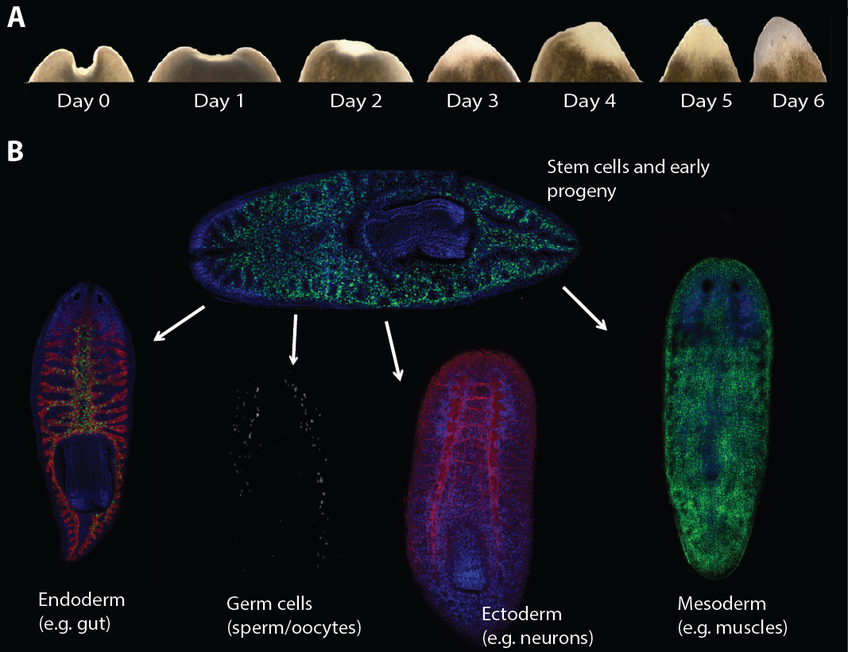This image is a scientific diagram on a black background, divided into two sections: Section A and Section B. 

**Section A**, positioned along the top edge of the image, reveals the daily progression of a small brown object from Day 0 to Day 6. On Day 0, the object has an indented center and rounded edges. It gradually transforms, and by Day 6, it develops into a claw-like shape. The object's growth stages are outlined clearly, showing its evolution over the span of a week.

**Section B**, situated below Section A, portrays various microscopic entities with vivid colors including green, blue, purple, and magenta. This section starts with a central, oval-shaped structure labeled "stem cells and early progeny." From this central structure, arrows extend to different shapes representing specific cell types: endoderm, germ cells, ectoderm, and mesoderm. The detailed drawings highlight their distinctive characteristics and roles, involving gut cells, neurons, muscle cells, and reproductive cells (sperm and eggs), captured as they would appear under a microscope. The detailed, bright illustrations enhance the understanding of stem cell differentiation and development.